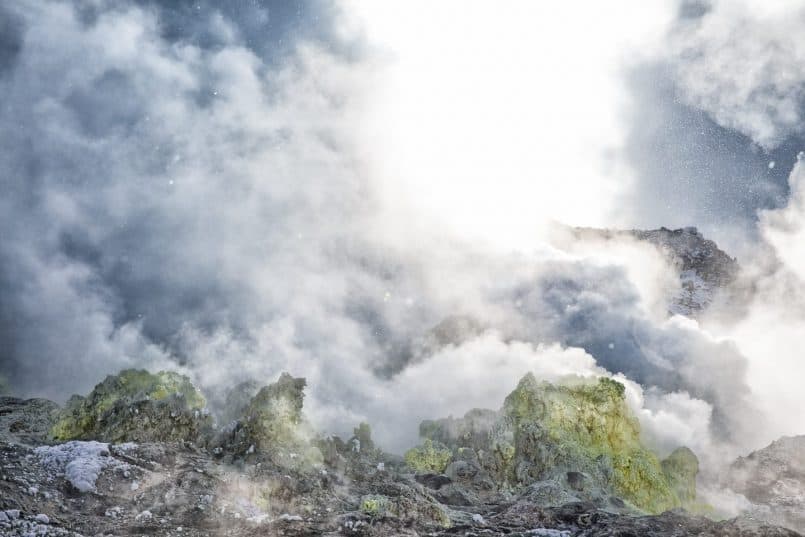This image captures a rugged outdoor scene dominated by dramatic natural elements. The foreground features a rough, almost rocky terrain in various shades of gray, with jagged green points that could be moss-covered rocks or possibly trees. This uneven ground is complemented by patches that might be snow or lighter-colored earth. Rising behind this foreground is what seems to be a further rock formation, suggesting a distant mountaintop.

The backdrop is enveloped by thick, voluminous clouds that range from pure white to dark blue, nearly gray, giving an impression of transition or impending weather changes. These clouds are especially dense and prominent, which hints at volcanic activity, as if a plume of smoke is being expelled from a hidden mountain. The sky beyond the clouds features a dark grayish-blue hue, intensifying the image's atmospheric tension.

Overall, the image is devoid of any visible human-made objects or text, focusing entirely on the natural setting. The earthy tones of the ground—including dirt, stones, and patches of grass—contrast with the expansive, cloud-filled sky that occupies the majority of the frame. This perspective suggests a high elevation, possibly looking up at a mountainous landscape under dramatic weather conditions.